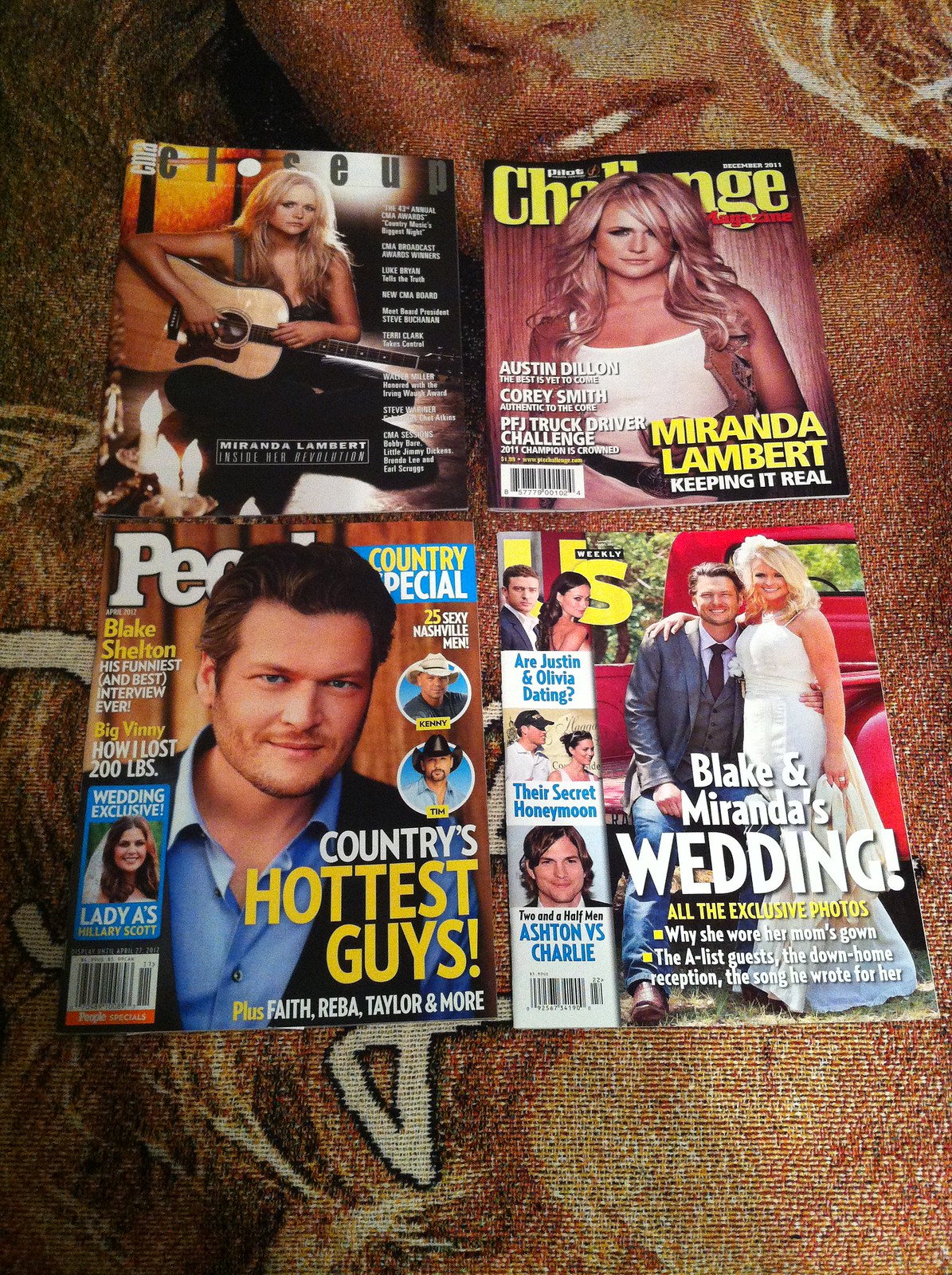This is a detailed top-down photograph of four popular gossip magazines, meticulously laid out on a patterned rug featuring a custom print of a woman's face. The magazines are arranged in a precise square formation, with two in the top row and two in the bottom row. In the top left corner, we have "CMA Close-Up" with Miranda Lambert gracing the cover. To its right is "Pilot Challenge Magazine," also featuring Miranda Lambert. On the bottom left sits "People Magazine," highlighting Blake Shelton with a prominent headline about the "Country's Hottest Guys." Completing the square on the bottom right, "Us Weekly" boasts exclusive coverage of Blake Shelton and Miranda Lambert's wedding, including exclusive photos and additional features like "Ashton vs. Charlie," a "Secret Honeymoon," and "Justin and Olivia." The arrangement of the magazines on such a distinctive rug makes for an eye-catching display.